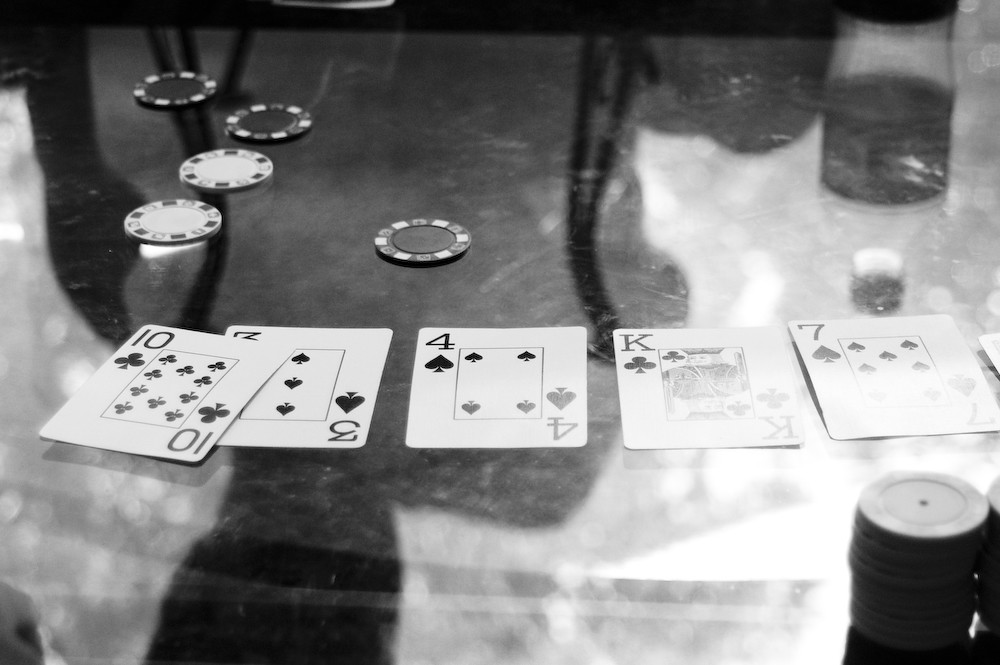The black and white image captures a moment of intense focus and anticipation at a card table. Though the image is slightly grainy, it clearly depicts a highly polished surface that reflects the silhouette of a person leaning over it, perhaps deeply engaged in a card game. On the table, five cards are meticulously laid out in a single row. From left to right, these cards are the 10 of Clubs, the 3 of Diamonds, the 4 of Diamonds, the King of Clubs, and the 7 of Spades. Scattered around the cards are several gambling chips, adding an authentic touch to the scene. The shimmering reflection of the person and the detailed arrangement of the cards and chips create a captivating composition, capturing a fleeting but revealing moment in a card game.